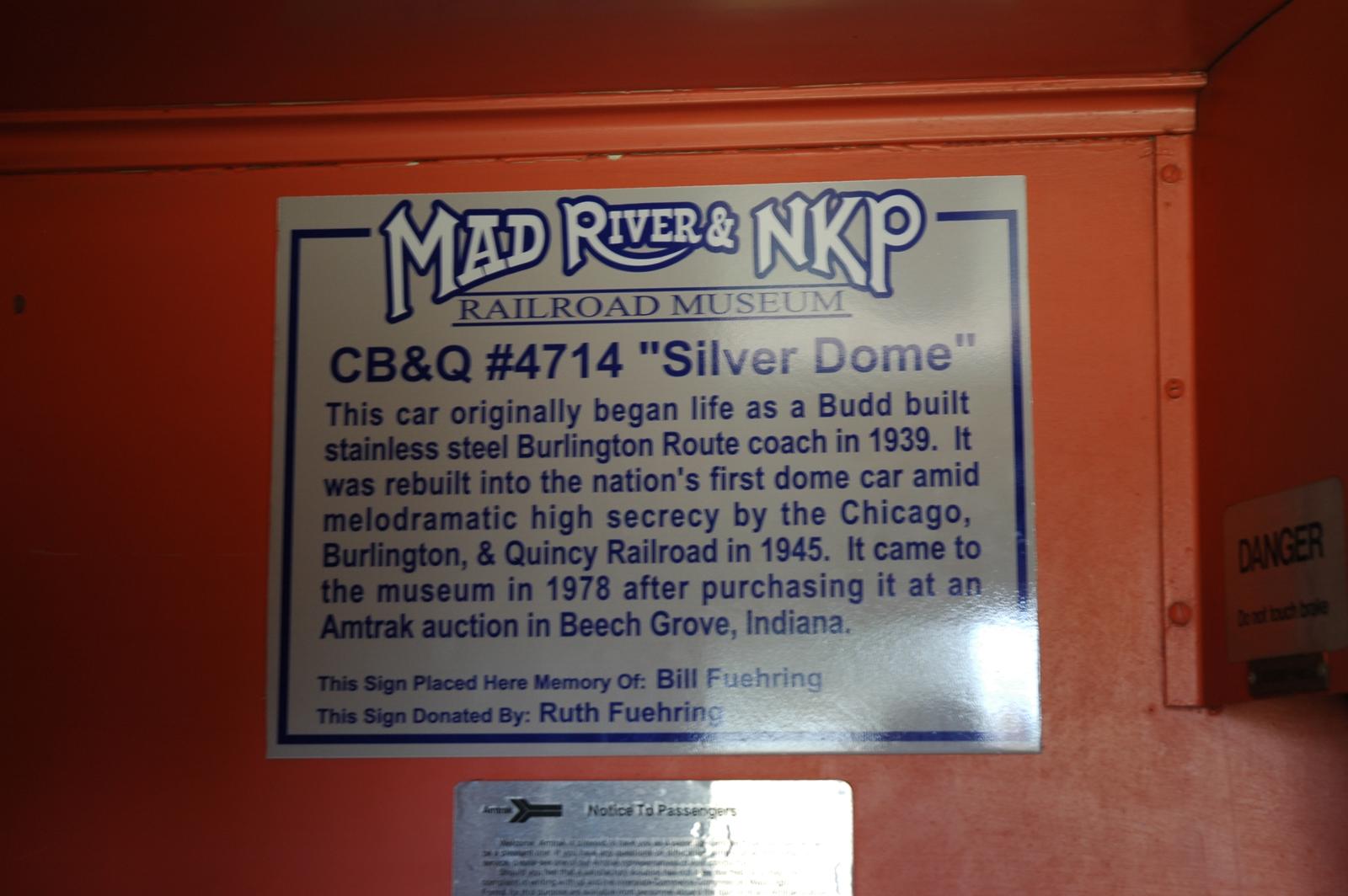The image features a vibrant fire engine red metal background with a detailed gray and silver plaque affixed to it. The main sign is inscribed with white and navy blue text and reads "Mad River and NKP Railroad Museum, CB&Q Number 4714, 'Silver Dome.'" This railroad car, originally a Budd-built stainless steel Burlington Route coach from 1939, was uniquely rebuilt into the nation's first dome car by the Chicago Burlington and Quincy Railroad in 1945 amidst dramatic high secrecy. It was acquired by the museum in 1978 through an Amtrak auction in Beech Grove, Indiana. The sign is dedicated to the memory of Bill Fuhring and donated by Ruth Fuhring. To the far right, partially obscured, there appears to be a metal sign indicating "Danger." Additionally, under the main plaque, there is a smaller sign labeled "Notice to Passengers," though its full text is unreadable.